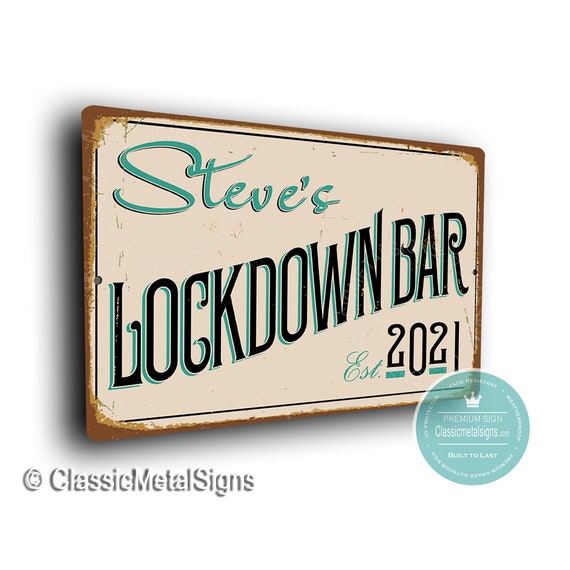This image features a vintage-style metal sign with a rusted, antique appearance along the edges. The rectangular sign has a creamy tan background with a black outline and depicts a mix of script and block lettering. At the top left in a stylized turquoise script, it reads "Steve's." Below, in bold black font with a teal drop shadow, it says "Lockdown Bar." The text "Established 2021" appears diagonally across the bottom right in a turquoise script. A watermark in white text at the bottom left corner states "Classic Metal Signs," indicating the manufacturer. On the bottom right corner of the sign, there's a circular seal with a crown logo, white text, and the phrases "Premium Sign ClassicalMetalSigns.com" and "Built to Last". The rust effect unifies the vintage aesthetic, giving the sign a weathered, nostalgic feel.